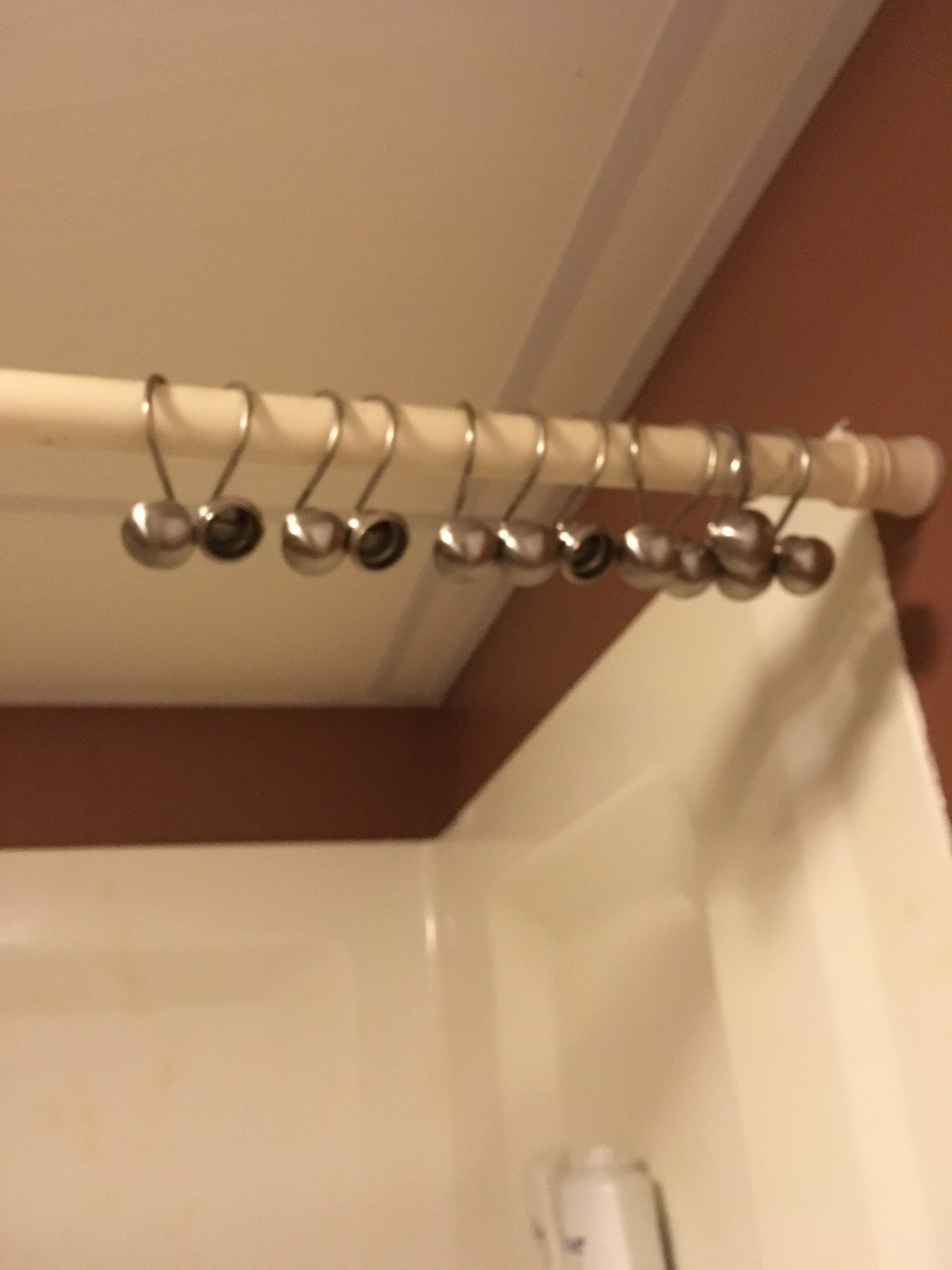The image depicts a somewhat blurry photo of a bathroom, mainly focused on a shower curtain rod and the metal hooks hanging from it. The shower rod, which is white, spans across the shower stall and holds eight silver metallic hooks, each designed with spherical, hollow balls. Although there is no shower curtain itself, the hooks are ready to hold one. The surrounding area includes a brown wall and a white ceiling with beveled edges, giving a contrast to the scene. In the background, white bottles of soap or shampoo are visible on a shelf inside the white-tiled shower stall. The overall color scheme of the bathroom showcases a blend of brown and white tones.